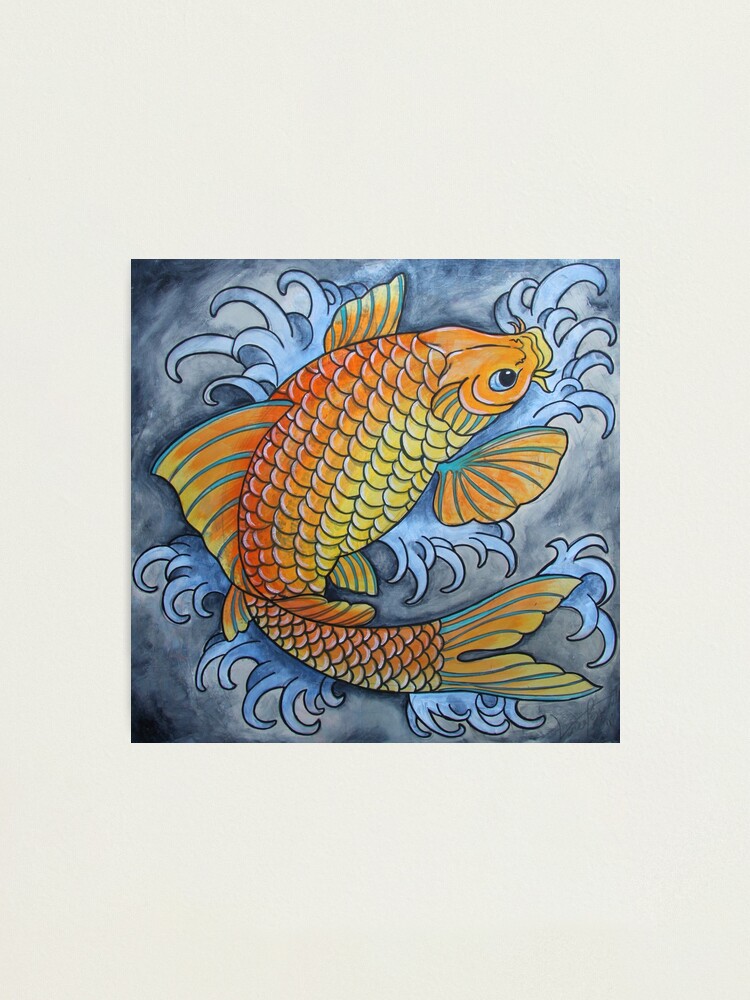This illustration, displayed within a neat white frame, features a vibrant and stylized depiction of a large orange and yellow fish, potentially a catfish or koi, illustrated with a gradient of gold, yellow, and orange hues. The fish's scales are especially prominent, resembling overlapping small axe heads, adding a unique texture to its body. Its blue eyes stand out along with its long, flowing fins. The fish is dynamically depicted splashing out of water, surrounded by swirling water in shades of dark to light blue. The background creates a dreamlike atmosphere with smoky, fluffy blue and light gray clouds, adding depth and contrast to the scene. Although there appears to be an artist's signature in the bottom right corner, it is not legible. The overall composition presents a whimsical yet detailed aquatic scene.